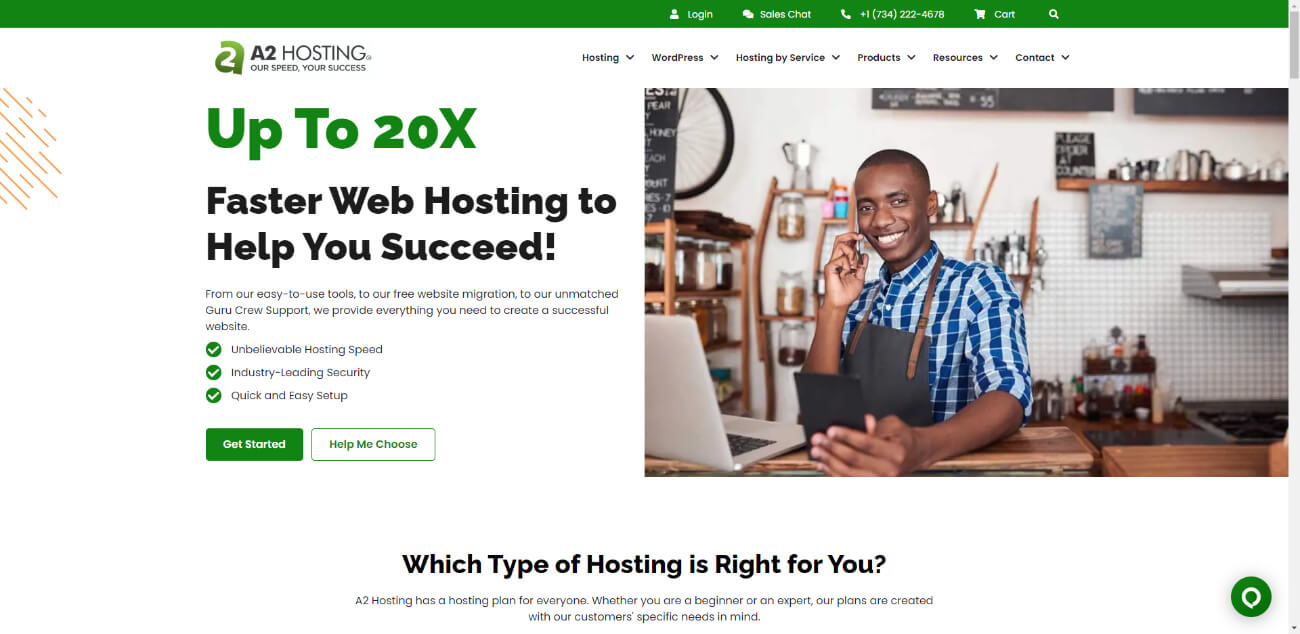The image portrays a sleek, professional website for a company called "2A Hosting" that specializes in internet or fast hosting services. Dominating the top of the page is a green banner featuring various navigational options, including "Log In," "Sales Chat," and a telephone icon next to the phone number "724-222-4676." Adjacent to these options is a shopping cart icon and a search bar for user convenience.

An eye-catching advertisement banner prominently displays the company's key selling point: "Up to 20x Faster Web Hosting to Help You Succeed." The "Up to 20x" text is highlighted in green, contrasting with the rest of the message in black for emphasis. Below this banner, there are interactive options highlighted in two chat bubbles—one green reading "Get Started" and another white reading "Help Me Choose."

On the right-hand side of the website, a comprehensive navigation menu lists various options, including "Hosting," "WordPress," "Hosting by Service," "Products," "Resources," and "Connect," offering users a broad range of services and resources. Additionally, the site features an image of an African-American male smiling while looking at his phone. He is casually dressed in a plaid shirt and is seated with a laptop, adding a relatable human element to the page.